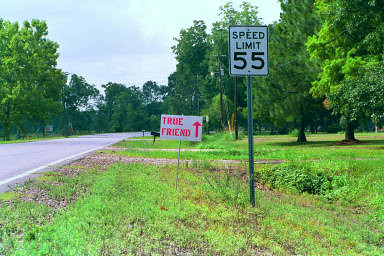In this outdoor daytime photograph, a side road meanders from the middle left to the distant center, lined with a mix of vibrant green grass and brown gravel in the foreground. Dominating the scene is a standard white speed limit sign perched on a green pole, explicitly stating "SPEED LIMIT 55" in bold black text. Closer inspection reveals a secondary sign slightly set back, mounted on a thinner gray pole. This sign features pink text and a pink arrow pointing upward, displaying the words "TRUE FRIEND." On the right side, a verdant canopy of trees begins to gather, while to the left, the road appears as a light gray ribbon winding away. Enhancing the scene are elements such as a black mailbox, followed by a white mailbox further back. Above, a sky with a gradient shift from grayish hues on the left to a clearer light blue on the right completes this picturesque setting.